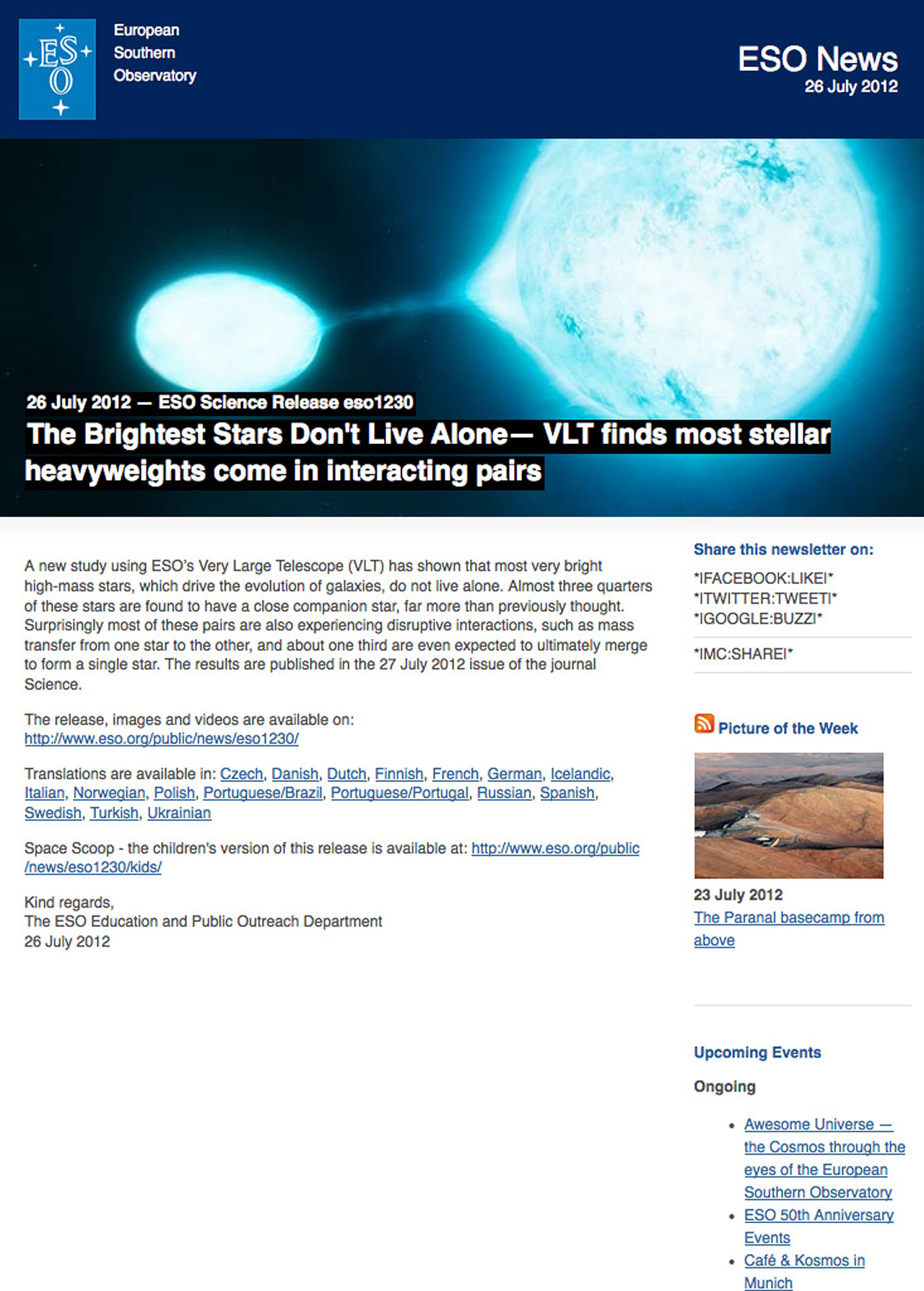**Descriptive Caption:**

"An image of an ESO News webpage dated July 28th, 2012. The top right corner of the page displays the date, while the top left corner features the ESO logo, a blue box containing the letters ESO with plus signs scattered around it. The logo stands for European Southern Observatory. 

At the center of the page is a large, dark blue photograph that prominently features two bright, connected circles with a glowing light blue around them. The accompanying caption reads, 'The brightest stars don't live alone. BLT finds most stellar heavyweights come in interacting pairs.' This visual representation underscores the finding depicted in the detailed paragraph that follows, explaining how a new study using ESO's Very Large Telescope reveals that most very bright, high-mass stars, which drive galaxy evolution, typically live in pairs rather than alone.

Below the paragraph, there is a clickable 'image release' link highlighted in blue. Additionally, the page provides multiple language options for readers, including Turkish, Polish, Danish, and Dutch, among others. The section concludes with 'Kind regards, ESO Education and Public Outreach Department.'

A 'Picture of the Week' segment showcases 'The Paranal Base Camp from Above,' featuring an image that intriguingly resembles a sea creature."